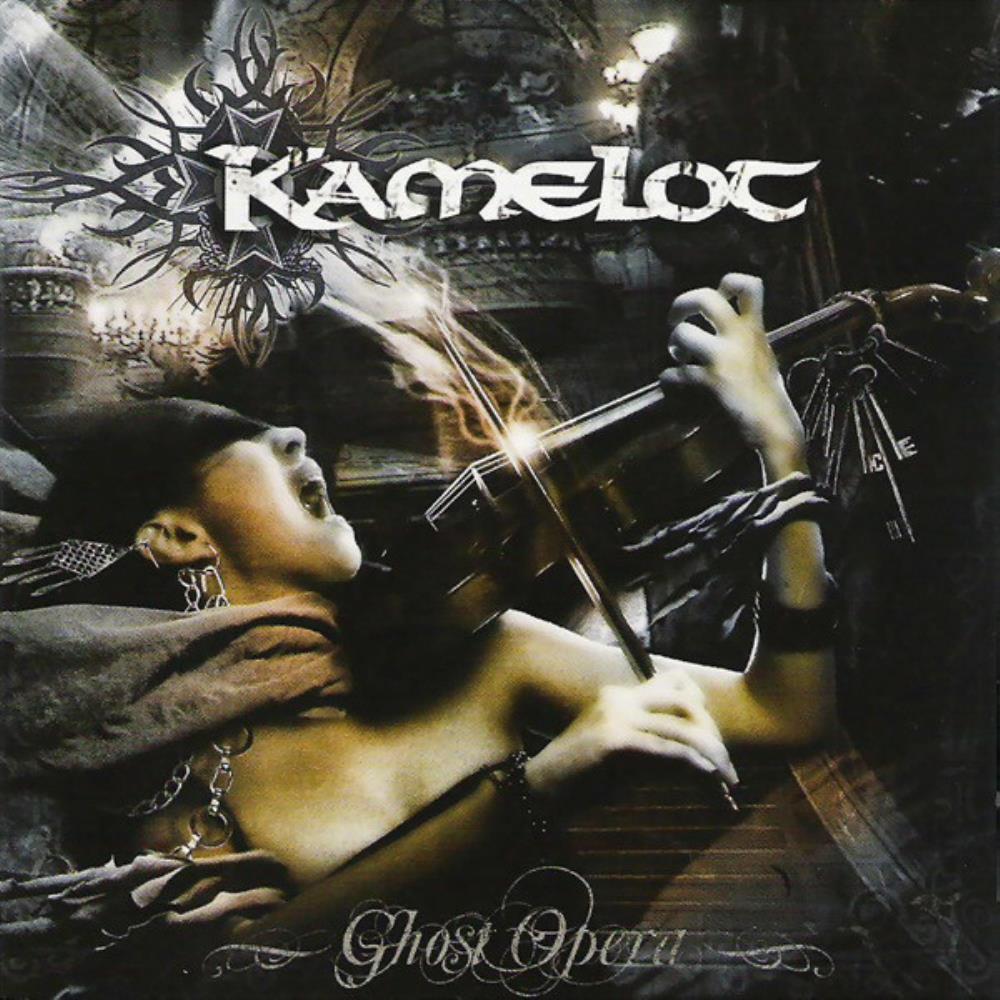The image portrays a dark, digitally altered scene resembling both an album cover and a movie poster. It features a distraught woman intensely playing a violin, which appears almost entangled with her. She has her mouth wide open, with her head thrown back and eyes covered in shadow, contributing to an expression of anguish or deep concentration. Her right hand holds the bow while her left hand presses the strings. Intriguingly, the violin has several keys hanging off it, and glowing smoke emanates from the instrument. She is adorned with long, chain-like earrings that sweep to the left, suggesting movement or a strong wind. The setting looks like an old, dilapidated theater with balconies, adding to the eerie atmosphere. The top of the image features the word "Camelot" in a bold, black, Gaelic-styled font, while the bottom displays "Ghost Opera" in Gothic cursive.